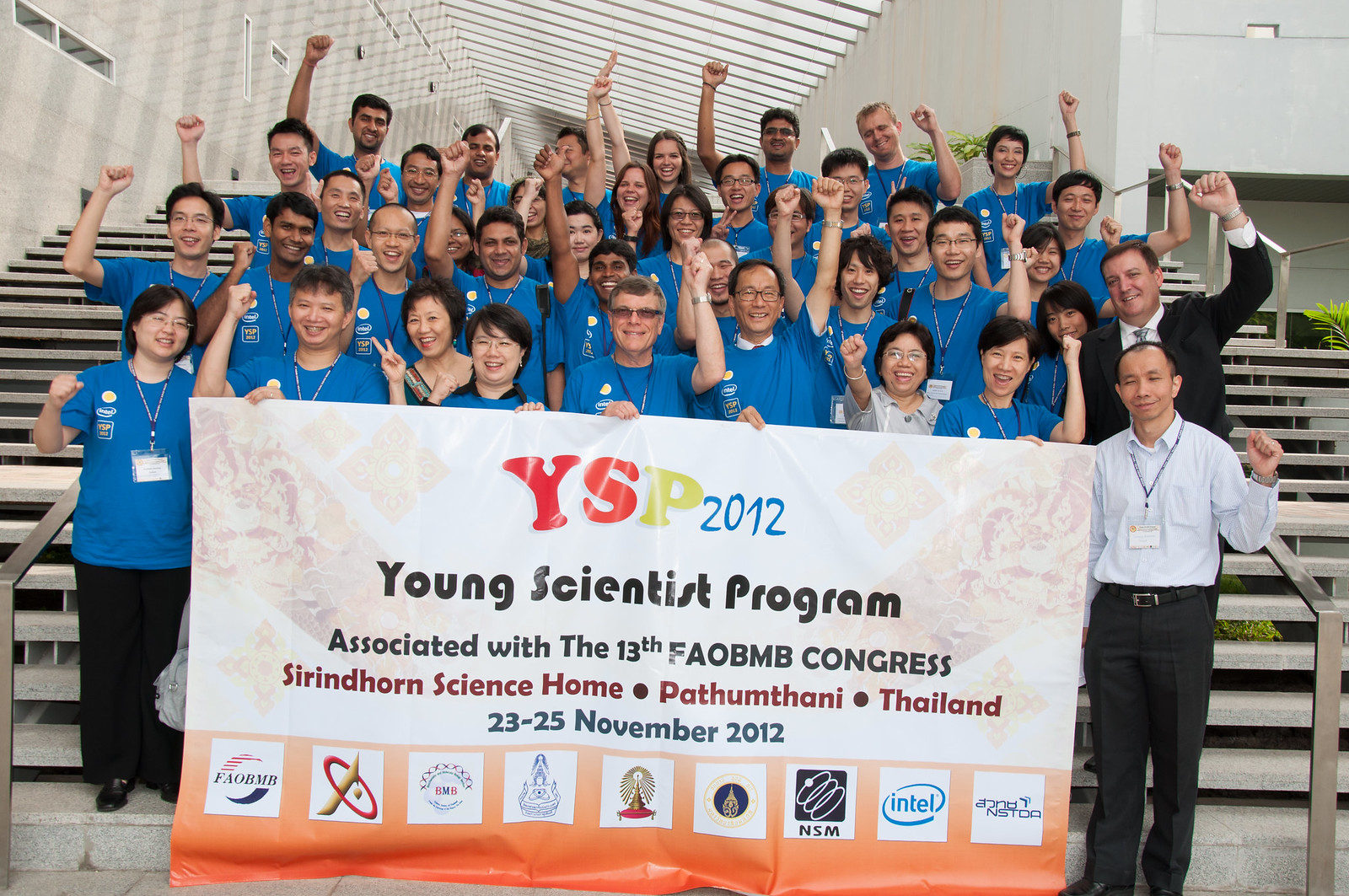The image captures a large, vibrant group of people standing on a broad, white concrete staircase with a modern white building as the backdrop. Most individuals are dressed in blue t-shirts featuring an indistinguishable logo on the chest. They are arranged in staggered rows, making every person visible at differing heights. The group members, smiling and exuding joy, have their arms raised, with some displaying peace signs and others clenching their fists in celebration. Prominently displayed in the foreground are two individuals holding a large, white and orange banner that reads: "YSP 2012 Young Scientist Program, associated with the 13th FAOBMB Congress, Sirindhorn Science Home, Pathum Thani, Thailand, 23-25 November 2012." At the banner's bottom edge, a series of logos from various sponsors, including those of NSN, Intel, and FAOBMB, are visible. On the left side of the image, narrow windows accent the white building wall, while to the far right, a metal handrail and a lush green palm frond are visible.